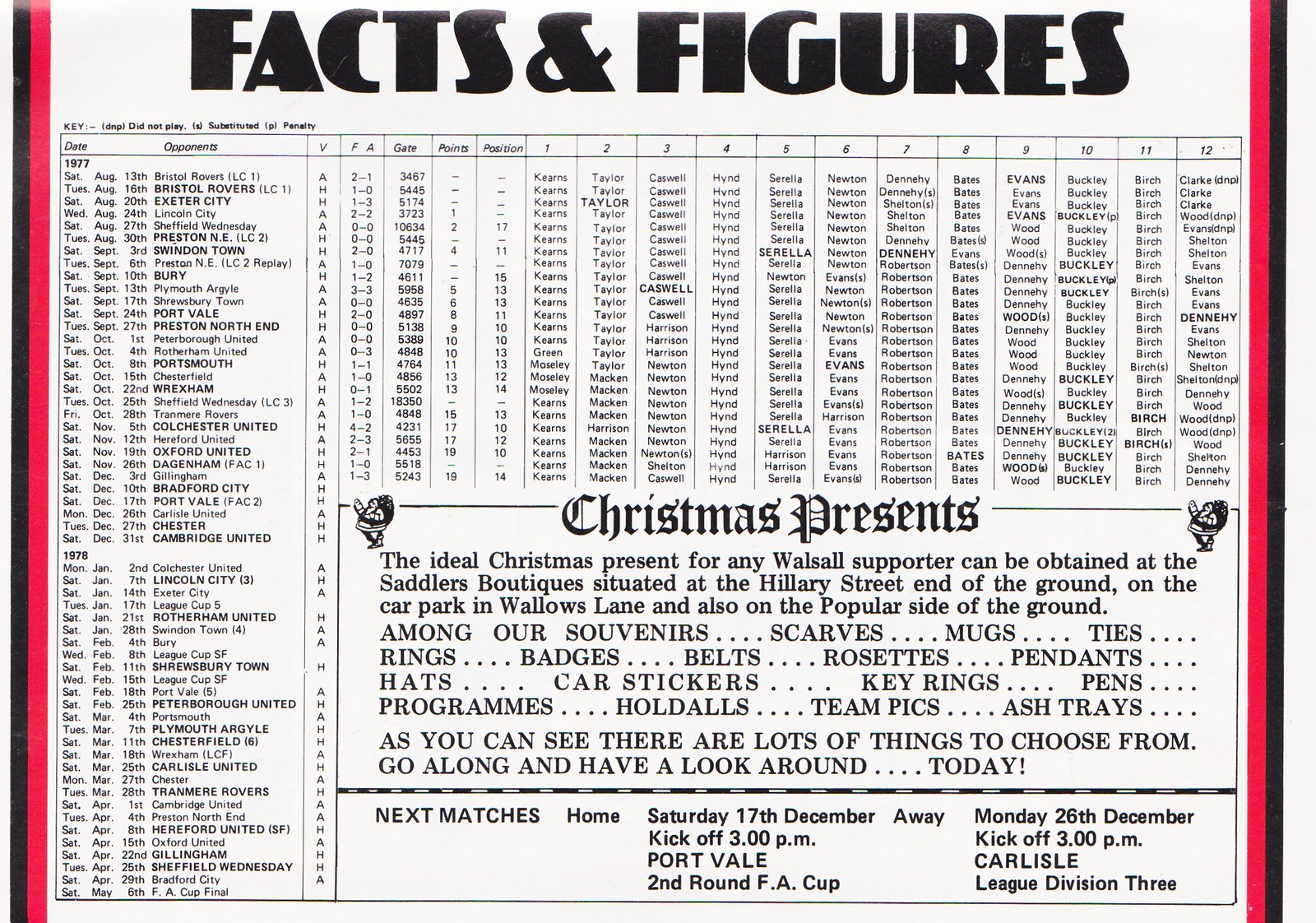This image is a densely detailed facts and figures sheet, bordered on the left and right by red, black, and white stripes. At the top, the title "Facts and Figures" is prominently displayed. The central section features a comprehensive chart listing dates and opponents from the 1977-1978 seasons, alongside columns detailing various match statistics, including a key for terms such as 'A' for substituted, 'P' for penalty, and 'DNP' for did not play. At the bottom, there's a dedicated section titled "Christmas Presents," advertising an array of Walsall F.C. memorabilia available at the Saddler's Boutique, located at multiple spots around their ground. Items listed for sale include scarves, mugs, ties, rings, badges, belts, rosettes, pendants, hats, car stickers, key rings, pens, programs, holla dolls, team pics, and ashtrays. The sheet also provides the schedule for upcoming matches, specifying home games, such as one on September 17th and away matches, including one against Carlisle on December 26th.